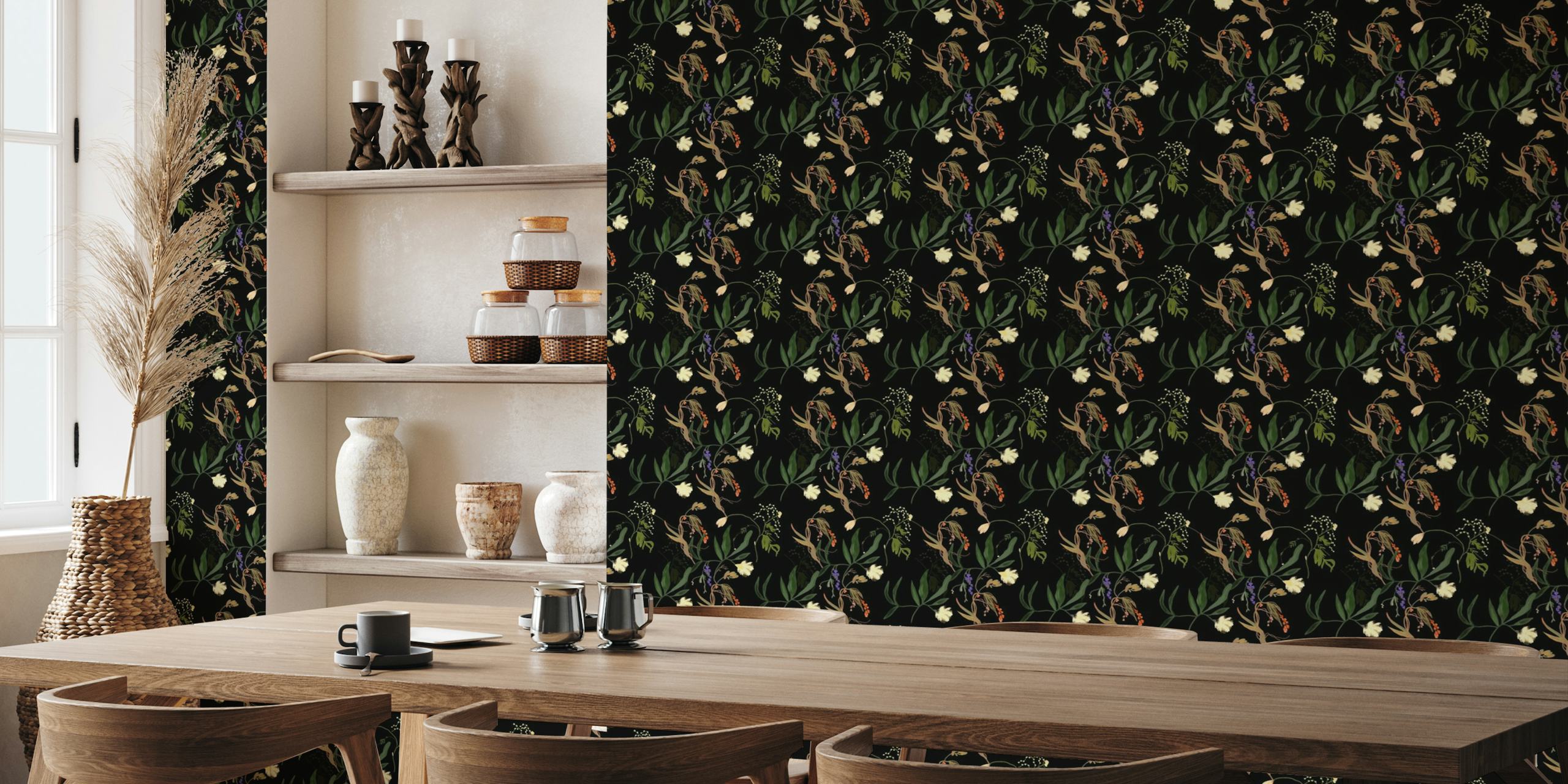The image captures a cozy yet sophisticated dining area within a home. Dominating the room is a large, light brown wooden table with a clean, rectangular shape, surrounded by six matching chairs. The table is adorned with various cups, lending a lived-in feel. A notable detail is a piece of paper on the table, adding a touch of everyday life. The back wall features a striking, mostly black wallpaper with a dynamic floral pattern, composed of white flowers, beige and dark green leaves, and subtle little dots of flowers, creating an eye-catching backdrop. 

To the left, there is a white shelf built into the wall, displaying an array of décor including brown candle holders, jars, and white vases, all contributing to the room's aesthetic. A window to the left allows natural light to flood in, enhancing the bright and welcoming atmosphere. The shelves also host candles, lamps, and several black mugs, adding contrast and depth to the setting. Overall, the arrangement and decor suggest a thoughtfully curated space that balances elegance with warmth.